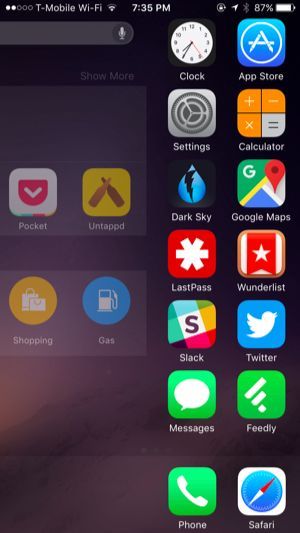This is a screenshot from an Apple device connected to the T-Mobile network. The status bar at the top displays "T-Mobile Wi-Fi" with a medium Wi-Fi strength indicator, the time as 7:35 PM, and the battery level at 87%. The home screen is populated with various apps.

On the left-hand side, there are two columns of apps, each containing seven apps arranged top to bottom. The first column features:
1. Clock
2. Settings
3. Dark Sky
4. LastPass
5. Slack
6. Messages
7. Phone

The second column includes:
1. App Store
2. Calculator
3. Google Maps
4. Wunderlist
5. Twitter
6. Feedly
7. Safari

To the right side of the screen, there appears to be a separate section, possibly a folder, housing four items. The top row contains the Pocket and Untappd apps, while the bottom row has Shopping and Gas. The exact nature of this section—whether it is a folder or a unique designation—is unclear. The screen captures a well-organized layout of frequently-used applications, providing a glimpse into the user’s preferred tools and utilities.